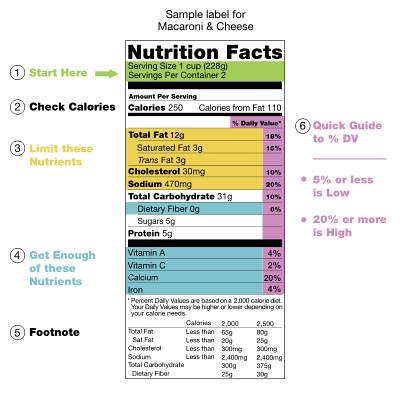This is a detailed image of a sample label for macaroni and cheese, structured as a vertical rectangular box outlined in black. At the top, it prominently reads "Nutrition Facts" with a white background. Beneath this, in a green section, it states the serving size (one cup) and servings per container (two). The label is divided by a thick black line, detailing the amounts per serving for various nutrients. 

Key areas include:
- **Calories**: 250
- **Total Fat**: 12 grams (including 3 grams each of saturated fat and trans fat)
- **Cholesterol**: 30 milligrams
- **Sodium**: 470 milligrams
- **Total Carbohydrates**: listed along with dietary fiber in a turquoise section.

Highlighted nutrients:
- **Dietary Fiber**
- **Sugars**
- **Protein**

A turquoise section details vitamins and minerals:
- **Vitamin A**
- **Vitamin C**
- **Calcium**
- **Iron**

Outside the main label, guiding instructions correspond with color-coded sections:
1. **Green**: Start Here – Serving Size and Servings Per Container.
2. **Black**: Check Calories – 250.
3. **Orange/Yellow**: Limit These Nutrients – Total Fat, Saturated Fat, Trans Fat, Cholesterol, Sodium.
4. **Blue/Turquoise**: Get Enough of These Nutrients – Dietary Fiber, Vitamins, Calcium, Iron.
5. **Black Footnote**.
6. **Purple**: Quick Guide to Percent DV – a guide indicating that 5% or less is low, 20% or more is high.

The entire image is neatly organized with color-coded sections to help identify key nutritional information, making it easier to understand what's beneficial or should be limited in the diet.